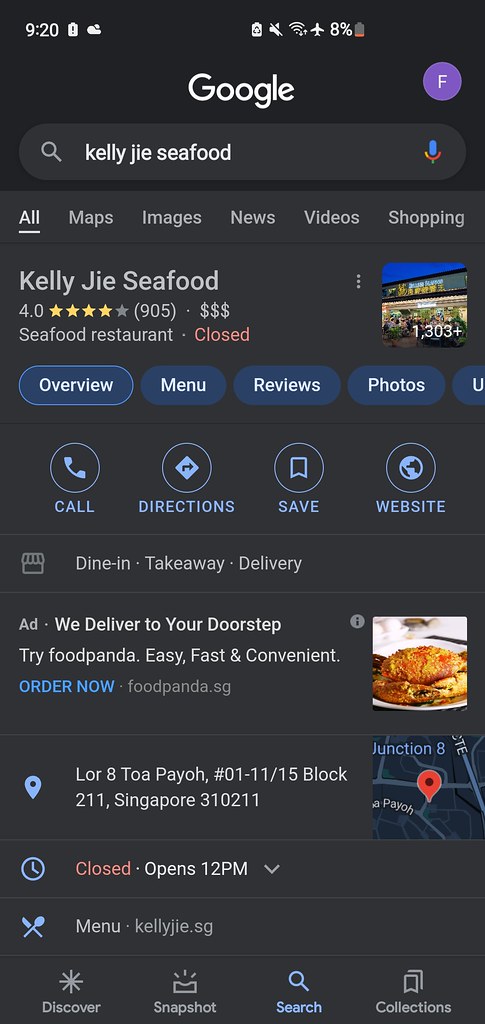This vertical image, taken from a smartphone, captures a Google search screen. The background transitions from a dull black at the top to a darker gray at the bottom. The top-left corner displays the time, 9:20, alongside various icons on the right, including a muted volume icon, Wi-Fi, airplane mode, and a battery icon showing 8% charge.

Central to the image is the Google search interface. The Google logo appears with a small, purple circle featuring an "F" to its right. Below this, the search bar contains the query "Kelly G seafood," accompanied by a microphone icon. The search options below highlight "All" and include Maps, Images, News, Video, and Shopping.

The search results reveal Kelly G Seafood is rated 4.0 stars based on 905 reviews, categorized as a $$ seafood restaurant, currently closed. Information available extends to tabs for Overview, Menu, Reviews, Photos, Call, Directions, Save, and Website, with services available for dine-in, takeaway, and delivery. A promotional message encourages users to order via Foodpanda for easy, fast, and convenient delivery. Additionally, the address and operational status of the restaurant are displayed, noting it is located in Singapore and opens at 12:00 PM.

Navigation options at the bottom of the screen show Discover, Snapshot, Search (highlighted), and Collections.